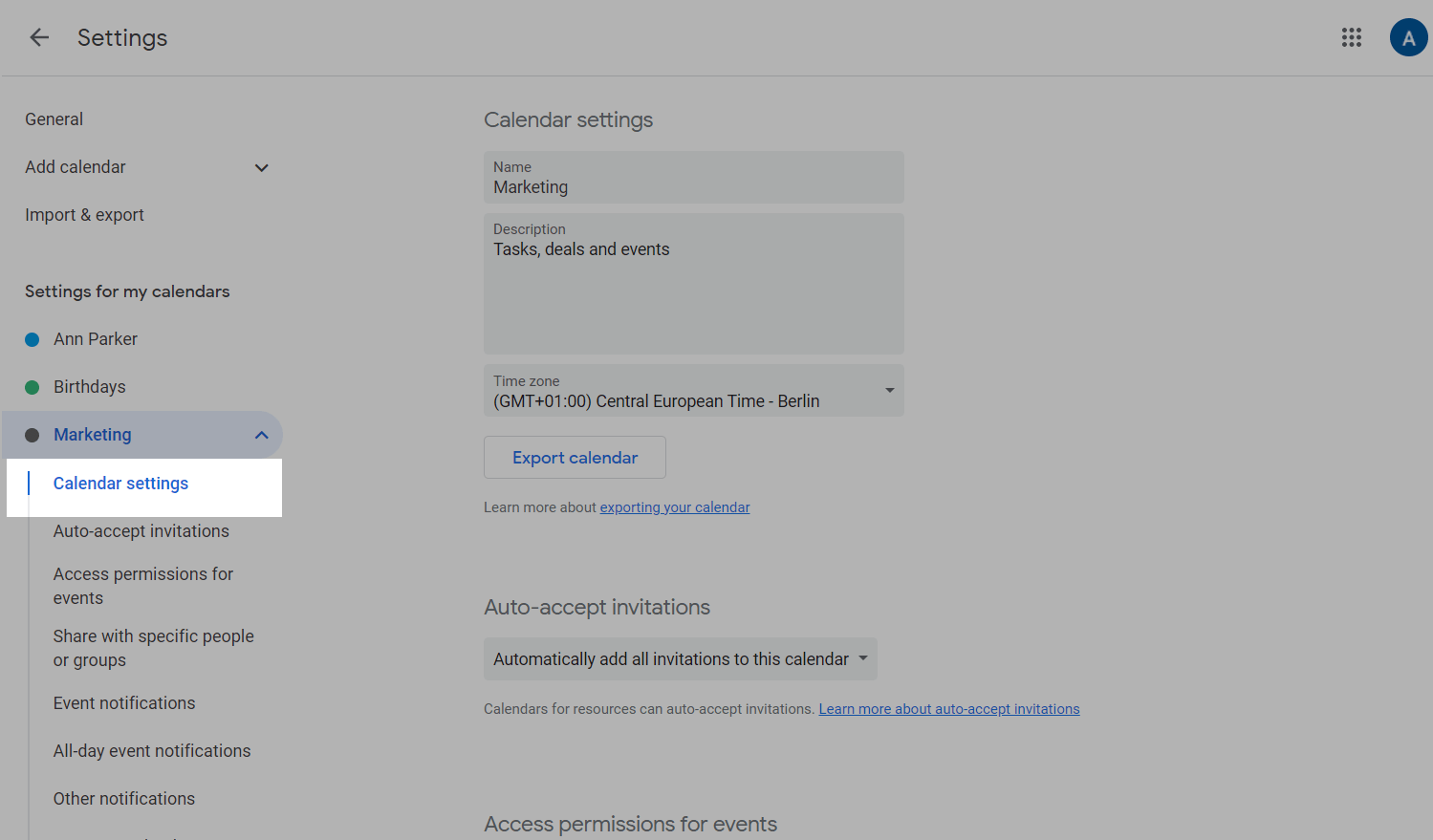The image depicts a gray-toned settings page of a calendar management website. In the upper left corner, the word "Settings" is displayed prominently. Directly adjacent to it, there's a leftward-pointing arrow that is very light gray, somewhat overlaying the text.

The page lists several options under a section that includes "General," "Add Calendar," and "Import and Export," followed by "Settings for my calendars." The user account or specific calendars listed include "Ann Parker birthdays marketing," with an additional drop-down menu indicated in blue text. 

Within a white bar labeled "Calendar Settings," there are options for "Auto-accept invitations," "Access permissions for events," "Share with specific people or groups," "Event notifications," "All-day event notifications," and "Other notifications."

Centrally positioned on the page, there are two main boxes under the "Calendar Settings" heading. One gray box is titled "Name Marketing," while the second box includes the categories "Tasks," "Deaths," "Deals," and "Events." Below this, there is an option to set the time zone, featuring a dropdown menu for selection.

Towards the bottom of the visible section, a blue box labeled "Export Calendar" offers export functionalities. Additionally, there are settings related to automatically accepting invitations, with the option to "Automatically add all invitations to this calendar," accompanied by another dropdown menu.

Further down, though partially cut off by the edge of the display, the website continues with settings for "Calendars for resources" and "Access permissions for events." A hyperlink labeled "Learn more about this" in blue text suggests additional information accessible by clicking. However, the full extent of options is not shown as the image cuts off at this point.